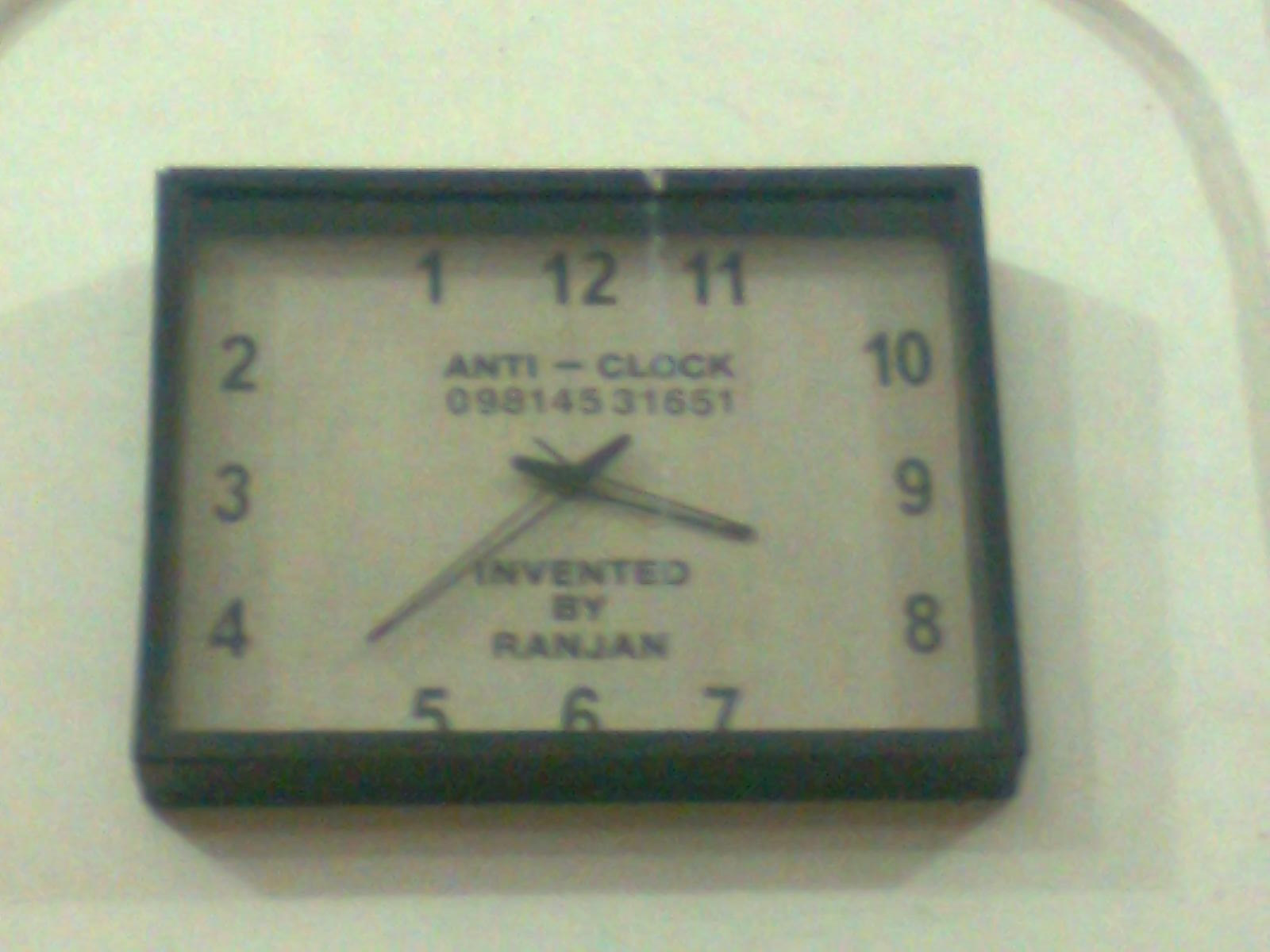This somewhat grainy image depicts a rectangular clock mounted on a wall inside a room with a white background that appears yellow under fluorescent or incandescent lighting. The clock is encased in a thick, likely wooden, black frame. Its white face bears the words "Anti-Clock" and the number "0981-453-1651" beneath it. Below the center, where the hands converge, it is inscribed with "Invented by Ranjan" with the name spelled out as "R-A-N-J-A-N." The clock hands are black with a white inlay and feature a very short second hand. Unusually, the clock runs in reverse, with the numbers arranged counterclockwise. The 12 and 6 are in their standard positions, but the 11 is at the 1 o'clock spot, and the count continues down to 1 at the 11 o'clock position. The numbers appear in black and are positioned in rows or columns beside the frame.